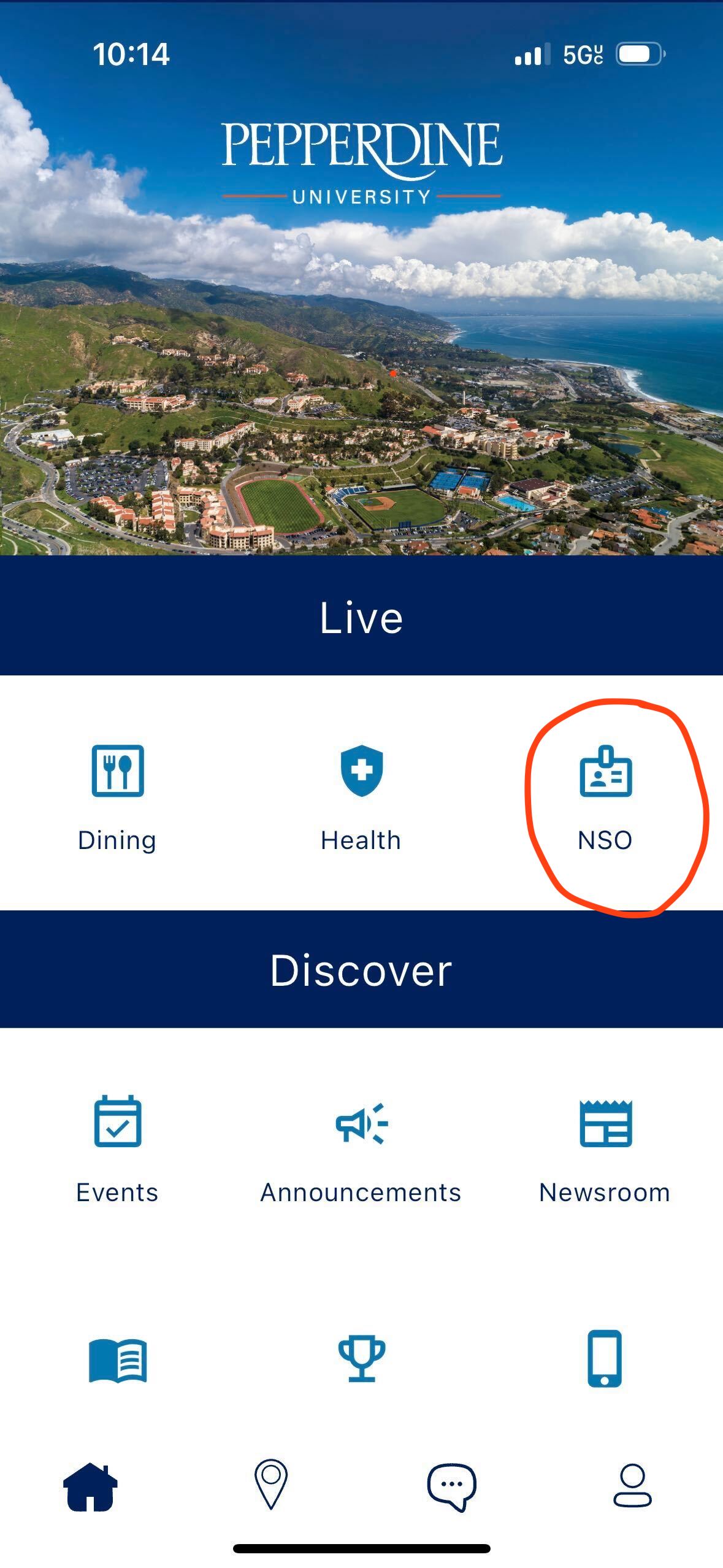This is a screenshot of a smartphone displaying the time as 10:14 AM. The battery icon shows it is about 80% charged, and the signal strength indicator shows three out of four bars. At the center of the screen, the words "Pepperdine University" are prominently displayed. The background image appears to be an aerial photograph, likely taken by a drone, showcasing a stunning landscape. The photograph features a vast blue sky with clouds clustered near the horizon. Below the sky lies a large body of water, a distant range of mountains, and a scenic coastline with a beach. In the foreground, there is a neighborhood populated with numerous houses, a football field, roads, and a baseball field.

At the bottom of the screen, there are several categories listed: "Live," "Dining Health NSO," "Discover," "Events," "Announcements," "Newsroom." Additionally, several icons are visible, including a book, a trophy, a smartphone, a home location pin, a text bubble, and a person icon. These icons likely represent different functions or sections of an app or interface related to Pepperdine University.